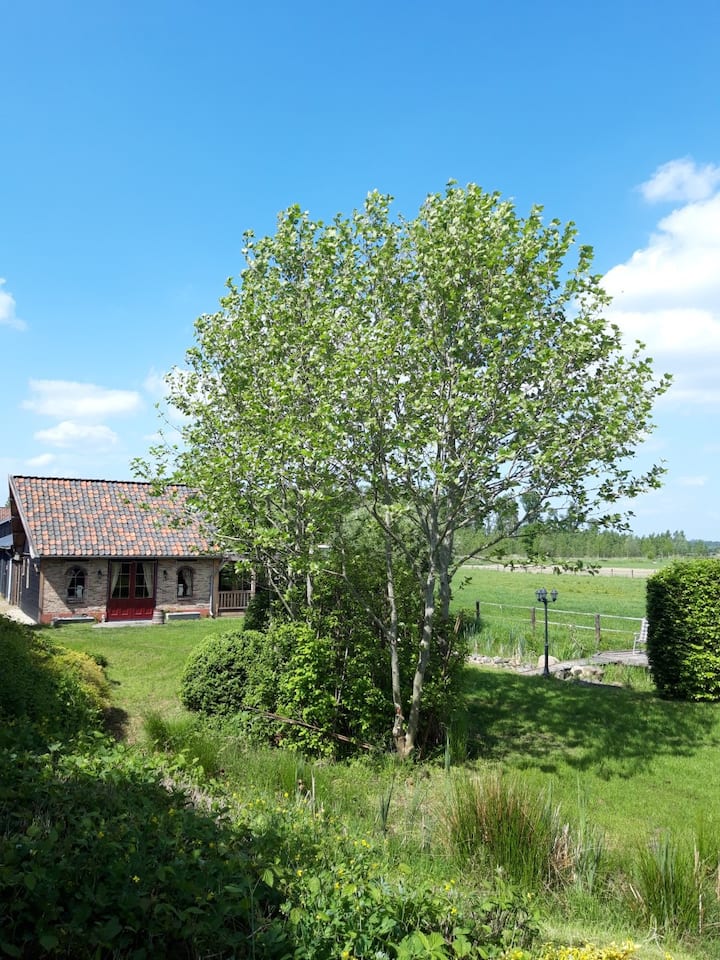The photograph, captured in portrait orientation, showcases a backyard of a small one-story brick house with a triangular roof composed of brown and black shingles. The house, located in the middle left of the image, features a set of double red doors with windows and curtains, flanked by two arched windows. The focal point of the image is a circular cluster of trees and bushes situated prominently in the center of the meticulously mowed green lawn. The trees are low with a rounded canopy of light green leaves. In the bottom left quadrant, the lawn transitions into an area of overgrown grass and weeds. Beyond the yard, on the right side of the image, a small wooden fence separates the yard from an expansive grass field that stretches into the distance, eventually meeting a forest on the horizon. Above, the sky is a clear light blue adorned with a few scattered white clouds, reflecting a bright, sunny day. The overall photograph is detailed and vertically oriented, emphasizing the serene and lush backyard scene.